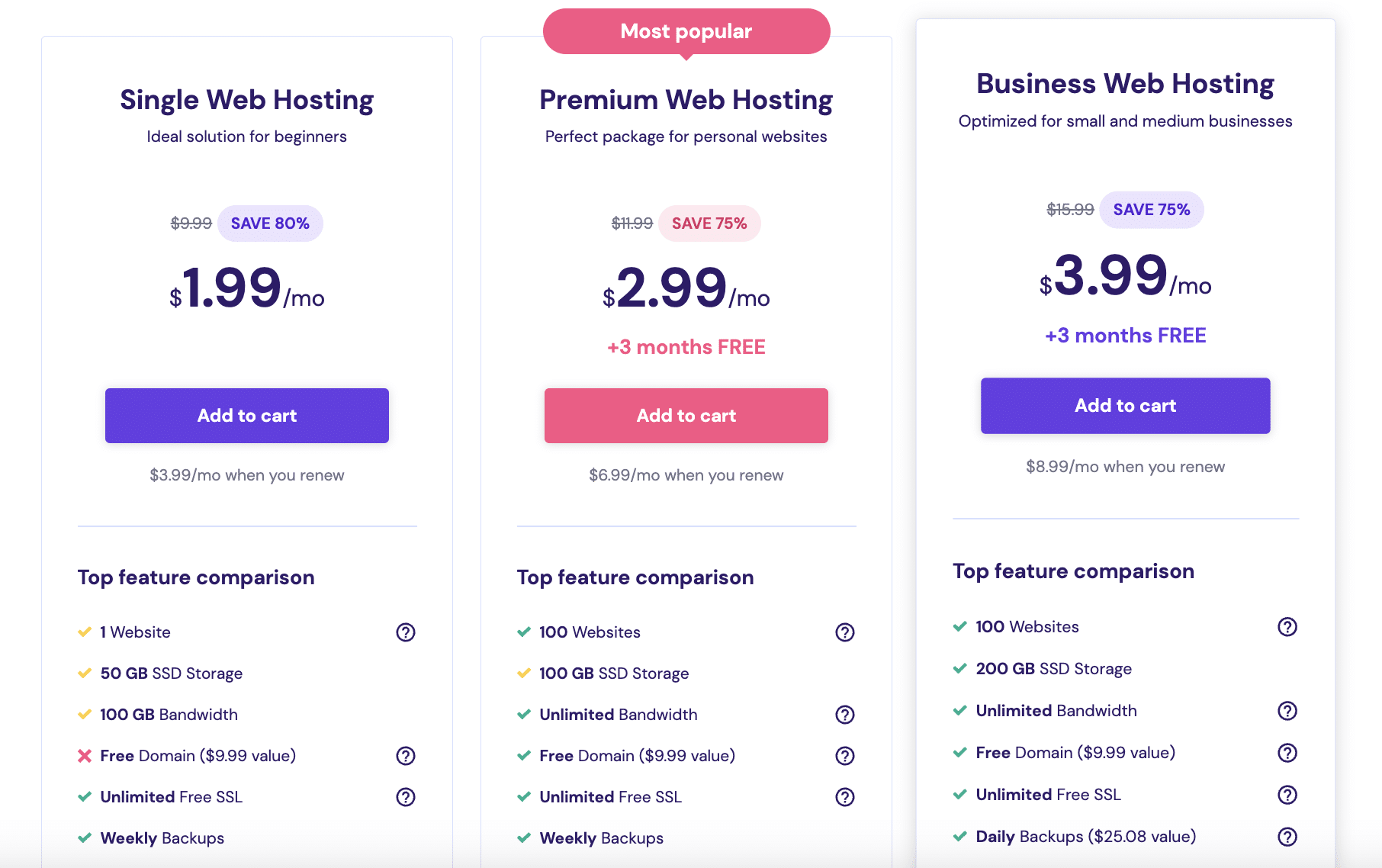This screenshot provides detailed information about three different web hosting options. 

1. **Single Web Hosting**:
   - **Ideal For**: Beginners
   - **Discount**: Save 80%
   - **Price**: $1.99 per month
   - **Add to Cart Button**: Available
   - **Top Features**: 
     - Hosting for one website
     - 50GB storage
     - 1GB bandwidth
     - Free domain (valued at $9.99)
     - Unlimited free SSL
     - Weekly backups

2. **Premium Web Hosting**:
   - **Ideal For**: Personal websites
   - **Discount**: Save 75%
   - **Price**: $2.99 per month, with an additional 3 months free
   - **Add to Cart Button**: Red and highlighted
   - **Top Features**:
     - Hosting for up to 100 websites
     - 100GB storage
     - Unlimited bandwidth
     - Free domain
     - Unlimited free SSL
     - Weekly backups

3. **Business Web Hosting**:
   - **Ideal For**: Small and medium businesses
   - **Discount**: Save 75%
   - **Price**: $3.99 per month

The screenshot emphasizes the most popular option, which is the Premium Web Hosting plan. Each option is designed to cater to different needs, with corresponding storage, bandwidth, and additional features tailored to help users decide the best plan for their requirements.